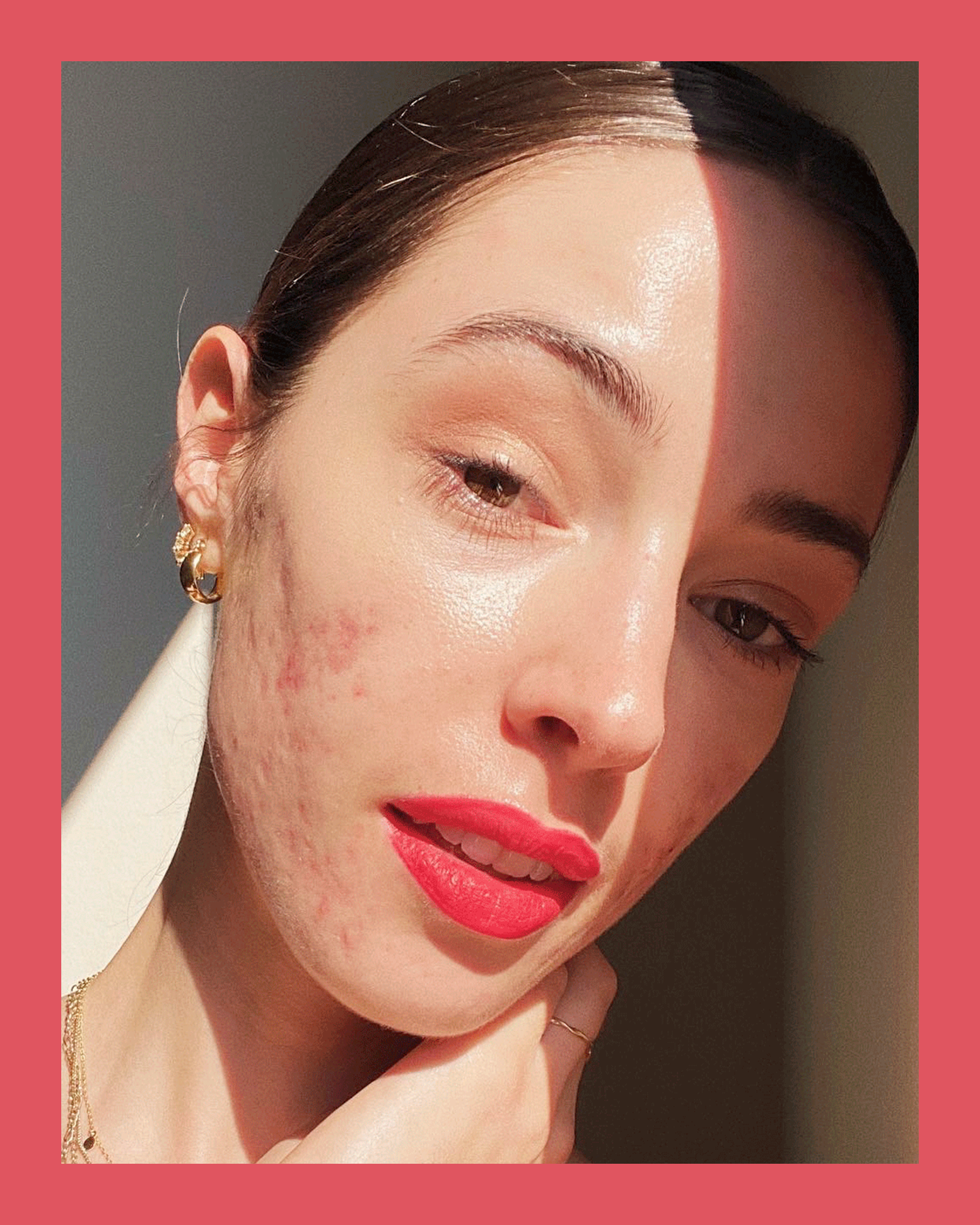In this realistic and close-up color photo, we see a woman with brown hair slicked back, creating a clean and polished appearance. Her face is partially turned, allowing the right side to be more prominent in the frame. Her brown eyes gaze directly at us, highlighting her perfectly geometric, clipped eyebrows that arch gracefully. She wears striking red lipstick, contributing to her composed and confident expression. Though she wears minimal makeup apart from the bold lipstick, her natural beauty is evident, with a slight smile revealing a glimpse of her teeth.

The woman rests her head against a white wall, and her right hand is positioned near her cheek. She accessorizes with at least one noticeable gold earring and a delicate gold necklace, with a hint of these elegant pieces visible in the frame. Additionally, a simple gold ring adorns her left ring finger. Despite some visible acne scars extending from her ears to her cheek and chin, her skin appears glowing and healthy overall.

The image is framed with a pink or mauve border, adding a soft touch to the composition. Overall, the captivating and detailed portrayal of the woman communicates a blend of strength and grace.